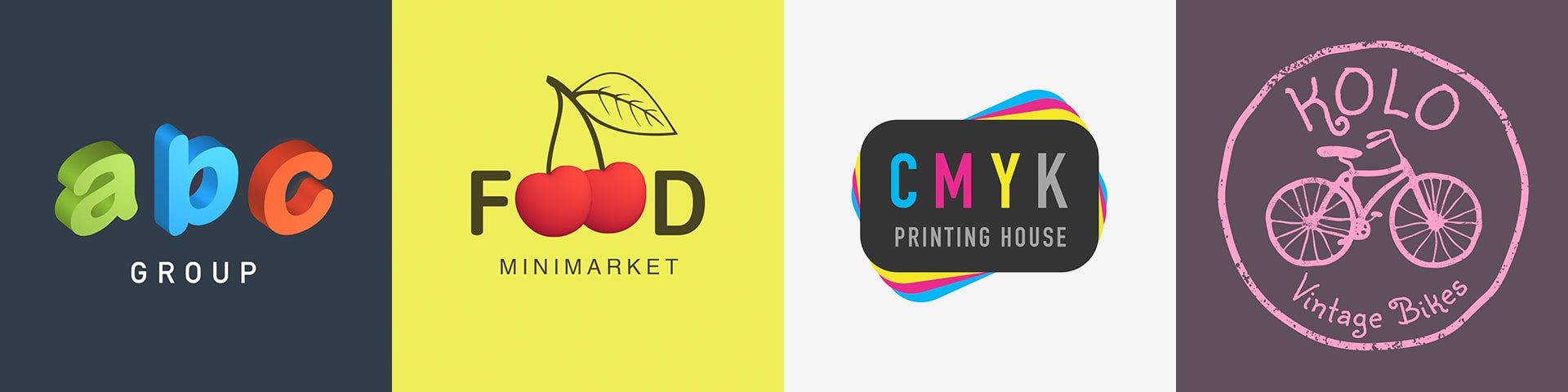This image displays a collection of four distinct logos or posters, each set within its own square frame. On the far left, against a navy blue background, the logo for ABC Group features three-dimensional letters: a green "A," a blue "B," and a red "C," with the word "GROUP" in white capital letters beneath them. Next to it, a logo with a yellow background showcases the word "FOOD," where the two O’s are artistically represented by red cherries connected by black stems and a leaf, accompanied by the text "MINI MARKET" in black capital letters below. The third logo, positioned on a grayish backdrop, belongs to CMYK Printing House and prominently displays the acronym "CMYK" with the letters colored in blue, pink (magenta), yellow, and gray respectively. The words "PRINTING HOUSE" are written in black underneath, and the design is framed by differently colored tags in the background. The final logo on the right features a purplish-blue-black background, centered with a pink circle. Inside this circle is the brand name "KOLO" in pink at the top, a side-view illustration of a bicycle also in pink, and the words "VINTAGE BIKES" at the bottom.